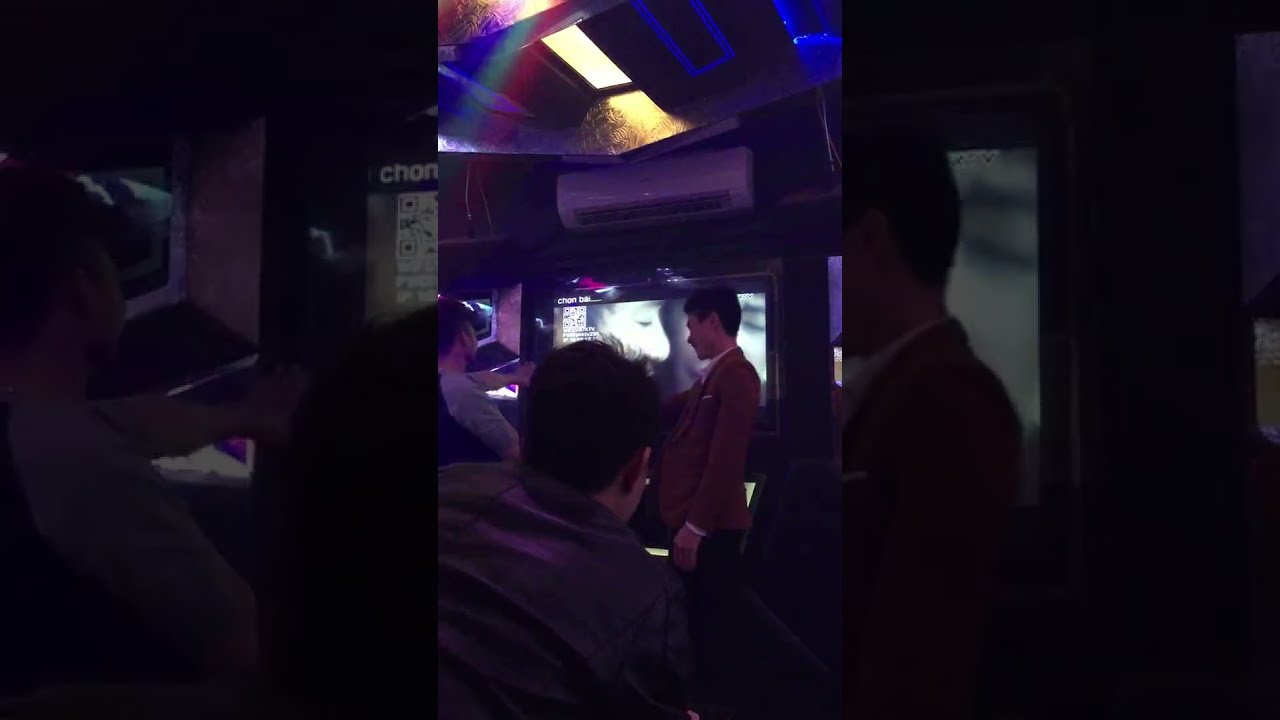The image is a horizontally aligned rectangular photograph with thick black borders on the left and right sides, creating a central focus on the picture. At the bottom center of the image, a man with short dark hair is partially visible, seen from behind and slightly to the left, wearing a dark, possibly green or gray shirt. The image captures him staring at a TV screen displaying two Asian men conversing, with subtitles in a language other than English appearing in blue and white. The TV screen occupies the middle panel of the photograph, flanked by black spaces on either side. Above the TV, a white horizontal AC unit is mounted on the wall. The room is mostly shadowed, with a dark ceiling adorned with blue-outlined bright rectangular lights and some yellow light filtering through. Overall, the setting appears muted and dimly lit, with the TV being the primary source of illumination.